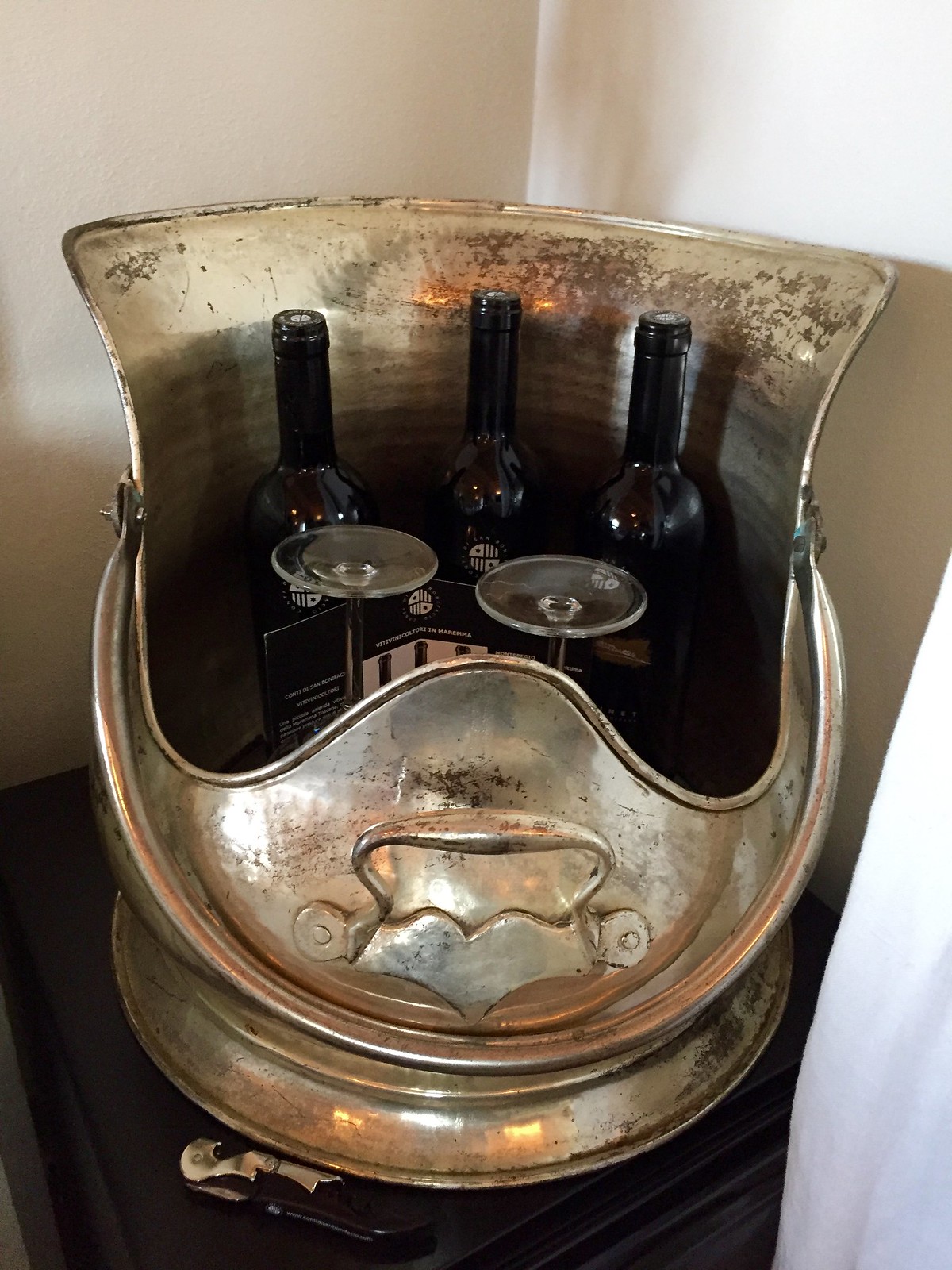In the corner of a room with off-white walls, a large metal container rests on a dark brown table, showcasing a meticulously designed bar setup. The container, resembling a grand urn or bowl with a brass lining around its upper edge, is primarily silver with visible areas where gold plating has worn away to reveal the brass beneath. This gives it an antique, well-used charm. A handle, hammered and riveted to the front, juts out slightly and doubles as a convenient grip.

Inside the container, three identical black bottles, likely wine, stand tall next to two upside-down wine glasses, their long stems and truncated bases distinctly visible. Adding to the display, a small black brochure peeks from within the arrangement. The entire assembly, including the table, appears elegantly set against the backdrop of off-colored white corner walls and a possible wooden floor, completing the scene with a touch of sophistication.